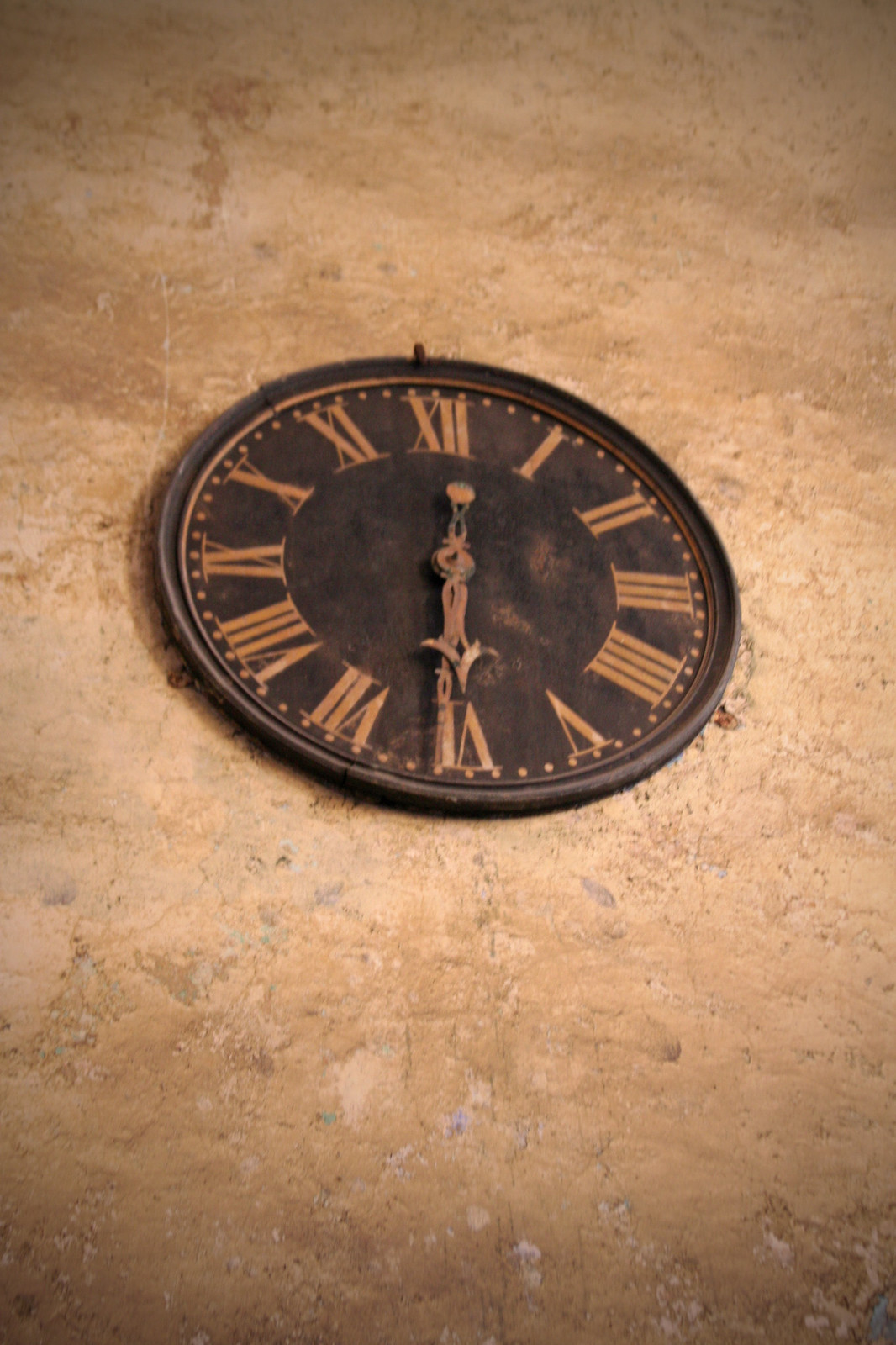The vertical rectangular image features an ancient, fancy analog clock positioned slightly above the center. The clock, which appears to be rusted and aged, hangs from a tab on a heavily weathered brown wall. The wall itself is marked with miscolored patches, stains, chips, and multiple long scratches. The clock face, made of black metal with brown Roman numerals in a dull, matte finish, contrasts the tarnished bronze or brass-like material surrounding the clock. The center of the clock is adorned with brown marks, further emphasizing its aged appearance. The corroded, somewhat rusty hands of the clock both point downward, indicating a time around 6:30. The perimeter of the clock face is decorated with small dots, adding to its vintage and ancient look.